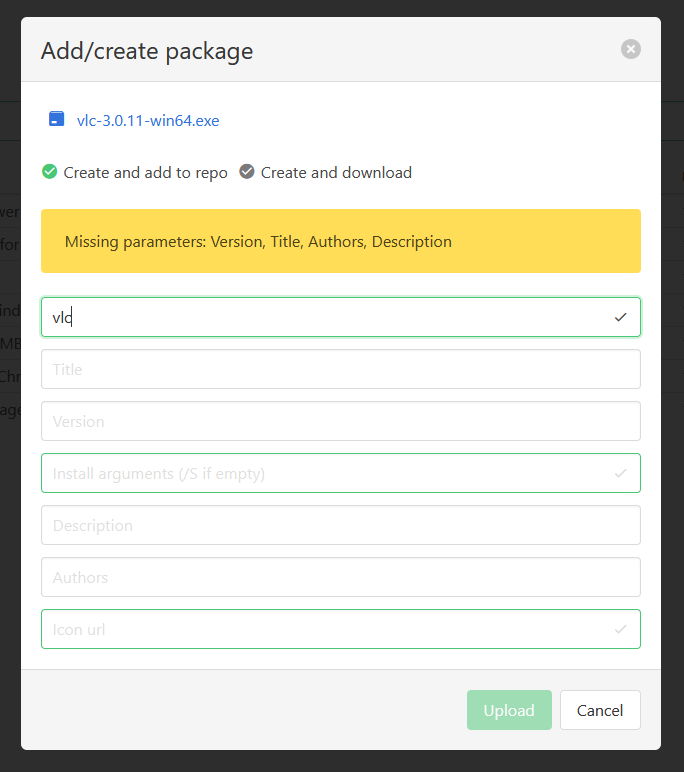This image is a screenshot depicting a software interface, likely a menu for creating or adding a package. The interface appears rectangular, with a black border framing the content. The central area of the menu is white and contains various elements organized in a vertical layout.

At the top, there is a title that reads "Add/Create Package." Below this title, there is an executable file listed, named "vlc-3.0-11-win64.exe." This file is presumably clickable and available for download.

Following the file listing, there are two buttons. The first button is green, featuring a checkmark, and is labeled "Create and Add to Repo." The second button is gray, also with a checkmark, and labeled "Create and Download."

Further down, there is a yellow notification bar displaying the message "Missing Parameters: version, title, authors, description." This indicates that some necessary information is yet to be provided.

Below this notification, there are eight text entry fields. In the first field, the text "VLC" has been entered, presumably as part of the package information.

Overall, the image appears to capture a step in the process of packaging software, highlighting both the fields required to complete the task and the options available for subsequent actions.